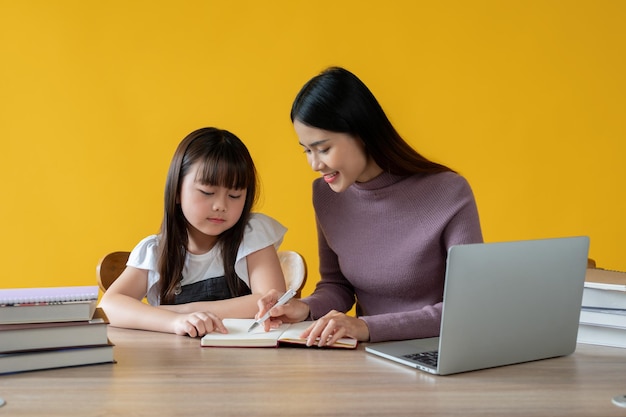This staged, stock-like photo captures a heartwarming scene of a woman helping a child with some work, possibly homework or a school activity. They sit at a light pine wood table set against a macaroni-colored background. The woman, of Asian descent, has long black hair and wears a light purple sweater or turtleneck. She holds a white pen in her right hand, pointing at something on an open book in front of her with a smile on her face. The child, also of Asian descent, has dark brown hair with bangs, and wears a white poofy-sleeve t-shirt with black overalls. The little girl sits to the left of the woman, mimicking her gesture by pointing at the same spot in the book. A gray unbranded laptop is positioned closer to the woman, angled toward her left arm. A stack of four to five books and a spiral notebook are arranged next to the laptop, and another stack of books with a notebook lies next to the child. The scene evokes a sense of focused and collaborative learning.